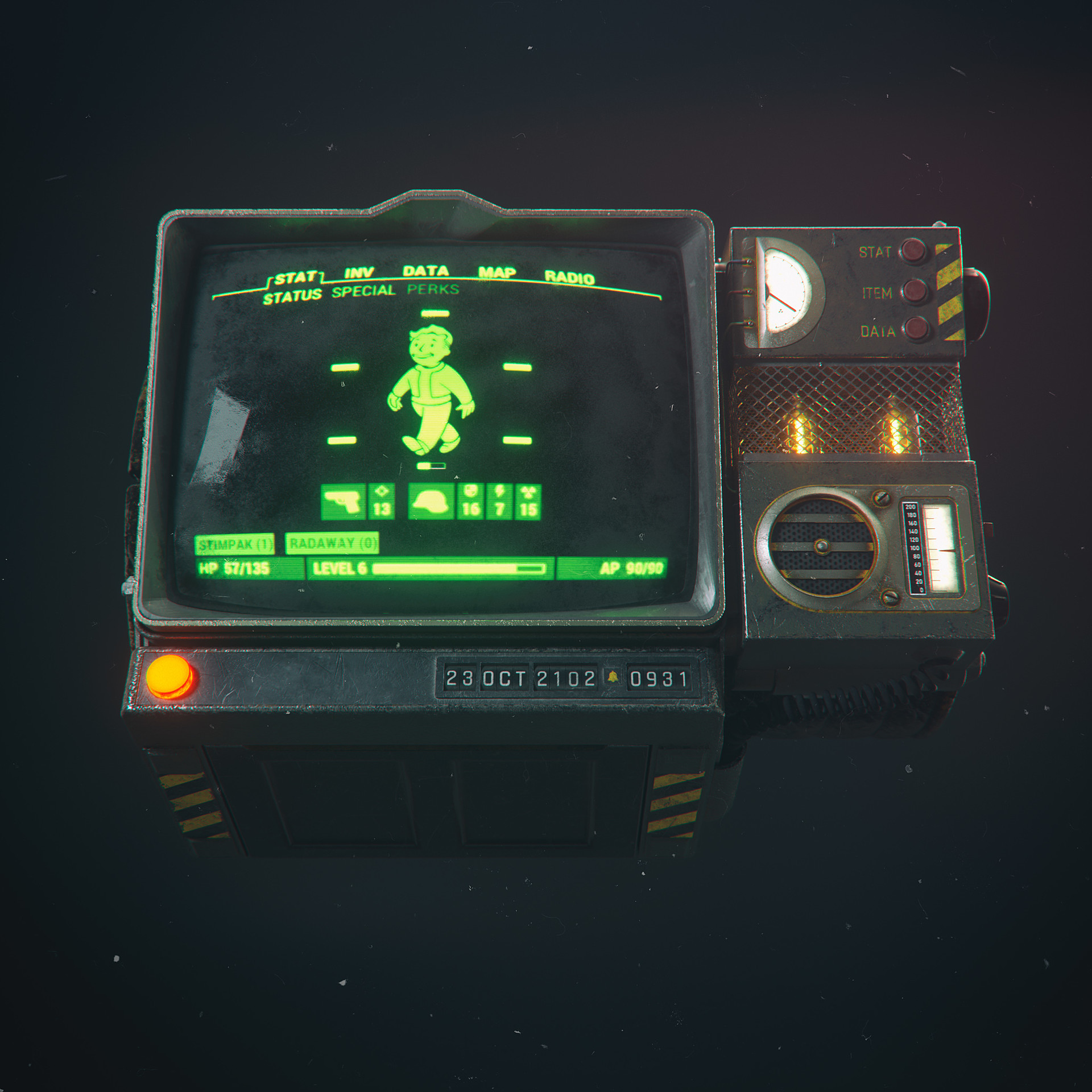The image showcases a meticulously crafted graphic artwork depicting a futuristic, metal-clad machine with a display screen at its center. The device, which evokes the retro design of an older television set or a time-traveling gadget, is set against a stark black background dotted with white stars, suggesting an outer space context. The main feature is the display screen, predominantly black, adorned with an intricate, green-tinted drawing of a boy. Encircling the boy, the screen displays various texts, such as "STAT," "INV," "DATA," "MAP," "RADIO," "STATUS," "SPECIAL," and "PERKS." Beneath this, some additional stats and an orange button are visible. On the right side of the machine, a cluster of round, red buttons labeled "STAT," "ITEM," and "DATA" are situated near functional meters. The gray metallic exterior with its futuristic design elements reflects heft and sophistication. Marked near the base of the machine is the date "23 OCT 21020931," further hinting at its futuristic origins. Overall, this image intricately blends elements of past and future technology, wrapped in a nostalgic yet advanced aesthetic.